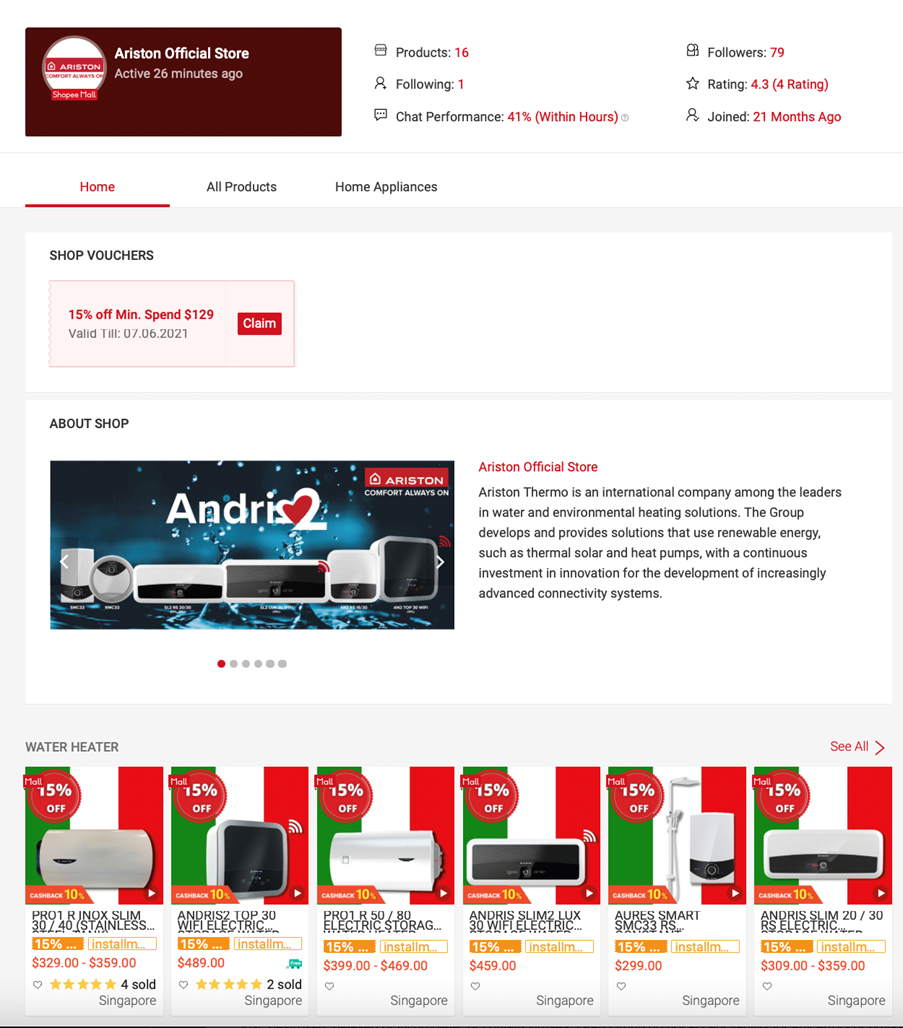This is a detailed description of a screenshot from the Ariston Official Store webpage:

The screenshot showcases the Ariston Official Store page, which appears to be part of an e-commerce platform. At the top, the store’s name is prominently displayed as "Ariston Official Store." The status indicates that the store was active 26 minutes ago. To the right, it shows that the store has 16 listed products, and it is following one person. The store's chat performance is rated at 41%, with "within hours" mentioned in parentheses. 

The store has garnered 79 followers and boasts a rating of 4.3 out of 5, based on 4 reviews. The store joined the platform 21 months ago. Below this information, there are tabs labeled "Home," "All Products," and "Home Appliances," with the current view being the "Home" tab. 

On this homepage, there is a section for shop vouchers offering "15% off on a minimum spend of $129," valid until July 6, 2021, with a red "Claim" button next to it. Under the vouchers, there is an "About Shop" section. This section includes a logo of Ariston and states: "Ariston Official Store - Ariston Thermo is an international company among the leaders in water and environmental heating solutions. The group develops and provides solutions that use renewable energy, such as thermal solar and heat pumps, with continuous investment in innovation for the development of increasingly advanced connectivity systems."

Further down, there is a display of water heaters, showcasing about six different products, with a "See All" option available.